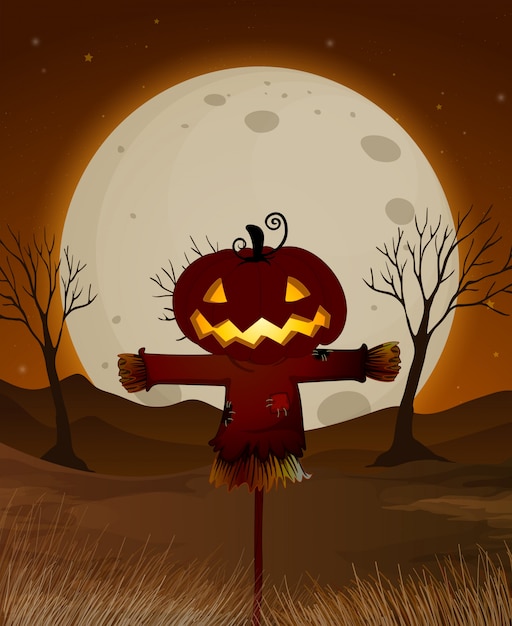The image is a 3D or AI-rendered illustration in portrait orientation, depicting a haunting scene of a jack-o'-lantern scarecrow mounted on a tall post in a barren field of beige grass. The scarecrow, centered in the image, is dressed in a long-sleeved tunic with bushy straw hands and legs, with its arms stretched out. Its head is a glowing, illuminated jack-o'-lantern featuring triangular eyes and a zigzag mouth, topped with a curly black stem.

The background showcases a dramatic night sky with an orange glow near the horizon that transitions to a deep burgundy color as it ascends. A full moon, occupying about two-thirds of the top part of the image, is prominent, displaying irregular gray craters and a white surface. Surrounding the field are three leafless trees, silhouetted against the moonlight, one on each side and one directly behind the jack-o'-lantern, enhancing the eerie atmosphere.

Additionally, the hill in the distance forms a dark brown silhouette against the sky. The color palette comprises shades of orange, brown, yellow, and black, creating a cohesive and spooky visual.